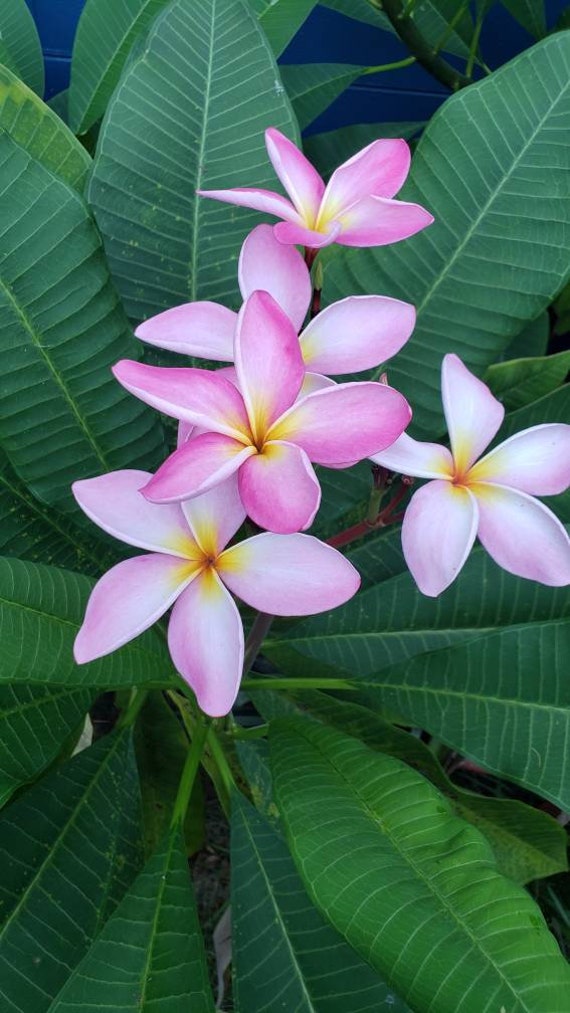The image depicts a vibrant and detailed scene featuring five pink orchid-like flowers as the focal point. These flowers, varying in shades from deep gradient pink to soft, nearly white pink, each possess five petals with distinct yellow centers that verge on orange. One flower even has a lighter, almost white hue. The flowers are set against a backdrop of lush, large green leaves resembling fern foliage, characterized by central veins that delineate the leaf structure. The flowers’ stems transition from red at the top to green as they reach the ground, suggesting the plant is rooted in soil rather than placed in a vase. In the far background, slightly visible, is a blue, possibly metallic object with a delineated line, which might be a car door or some architectural element. The overall setting appears to be outdoors, possibly in a garden, capturing the essence of nature’s vibrant beauty.